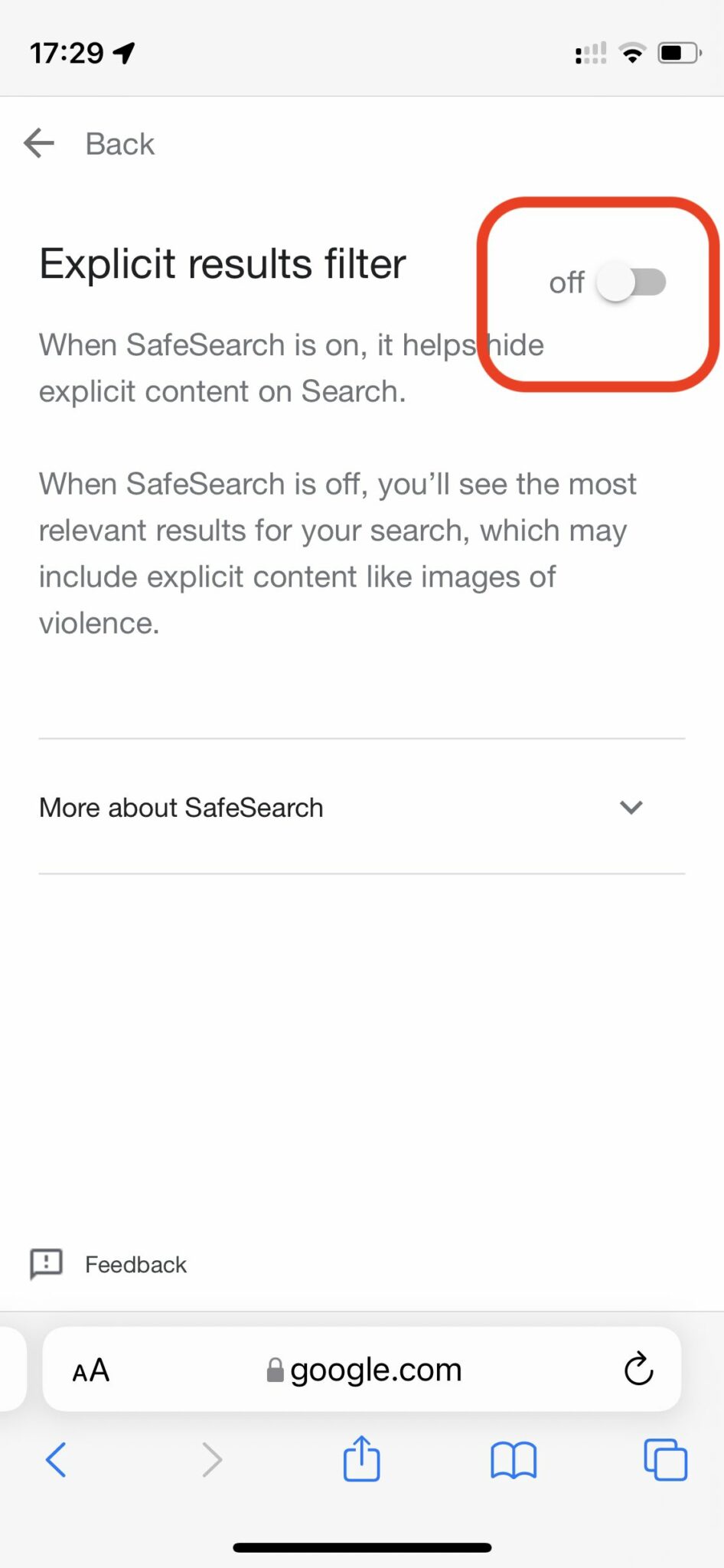The image features a white background with a timestamp of 17:29. At the top left, there is a back arrow icon. Below this, there is an 'Explicit Results Filter' toggle that is set to off, indicated by a red rectangle around it. When SafeSearch is enabled, it filters out explicit content from search results. When disabled, as shown in the image, the search results may include explicit content, including sensitive images. Below the filter toggle, there is a link labeled 'More about SafeSearch.'

On the right side, there are icons for providing feedback and initiating a chat, with the chat icon marked by an exclamation point. There are also text size adjustment options represented by a small 'A' and a large 'A,' and a 'google.com' URL is visible. Additionally, the interface includes a refresh icon, along with blue icons for navigation (left and right arrows), sharing (share icon), saving as a bookmark (book icon), and a display option (two overlapping squares).

At the bottom of the image, a solid black bar spans the width of the screen.